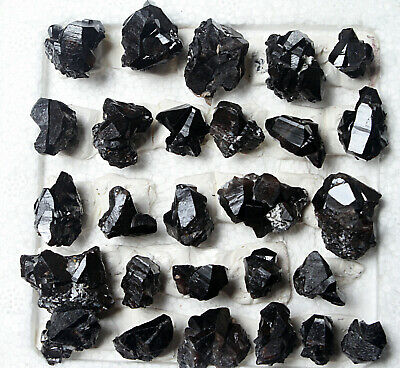A collection of black crystals of varying sizes and shapes are displayed on a white surface. The crystals include ovals, circles, and irregularly shaped triangles, with some appearing to incorporate smaller white crystals beneath them. The crystals are highly reflective, with light gleaming off their dark surfaces, revealing a rich assortment of hues. Close inspection shows layered patterns within the crystals, featuring shades of gray, white, and silver. The image quality is superb, with sharp focus and clear details, showcasing the shiny, mineral-like properties of the crystals. There are no additional objects or text in the image.